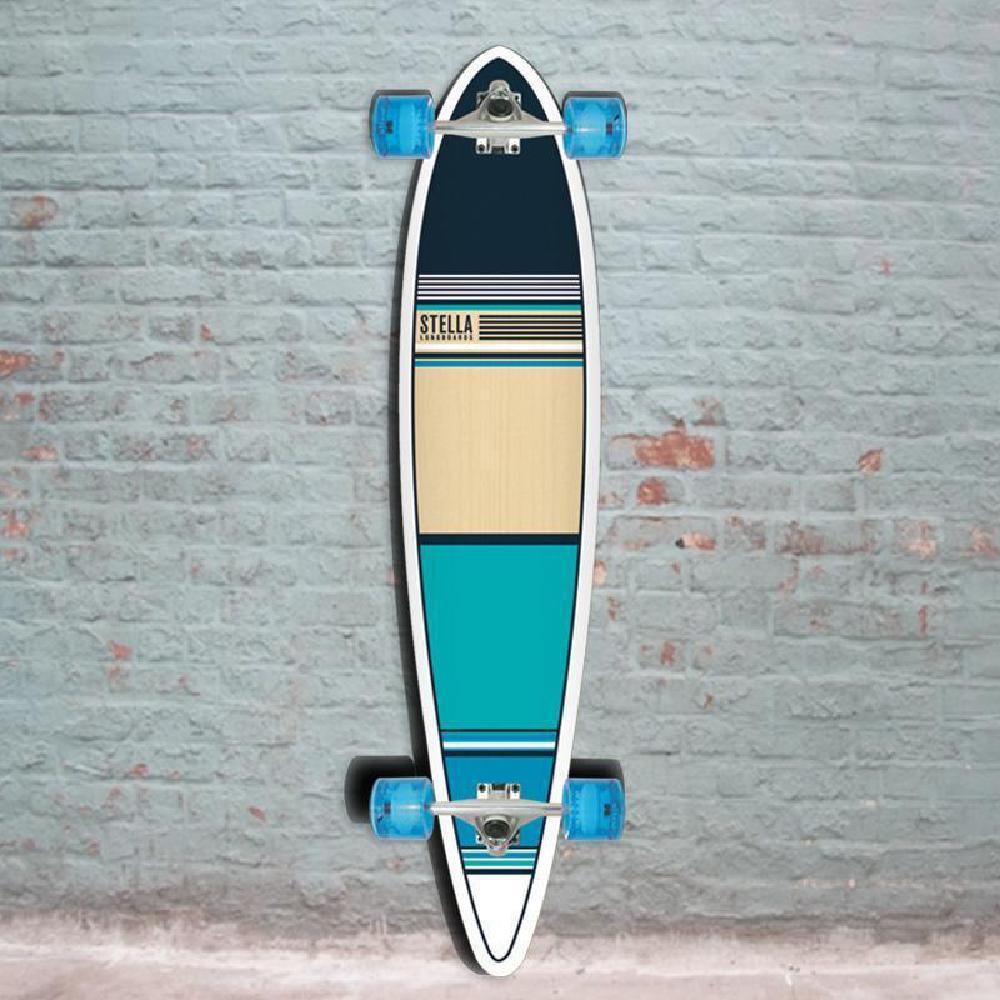This photograph features a longboard-style skateboard leaning vertically against a faded teal brick wall. The wall, with patches of red and white paint showing through, has a textured, weathered appearance. At the bottom, the wall transitions to solid white concrete. The skateboard, centered in the image and facing wheel-side out, boasts a visually striking design. It features an oval shape with pointed ends, trimmed with a white border. The deck is adorned with a geometric arrangement of colors and stripes: starting at the top with black, followed by horizontal black and white lines, transitioning to wood grain, then a thin black line, aqua, more lines, blue, and finally white at the bottom. The board also displays a logo with the word "Stella." The wheels are translucent blue plastic, adding a pop of color against the multi-hued backdrop of the wall. The photograph is a wide, vertical rectangle, capturing the skateboard in full detail along with the textured wall behind it.